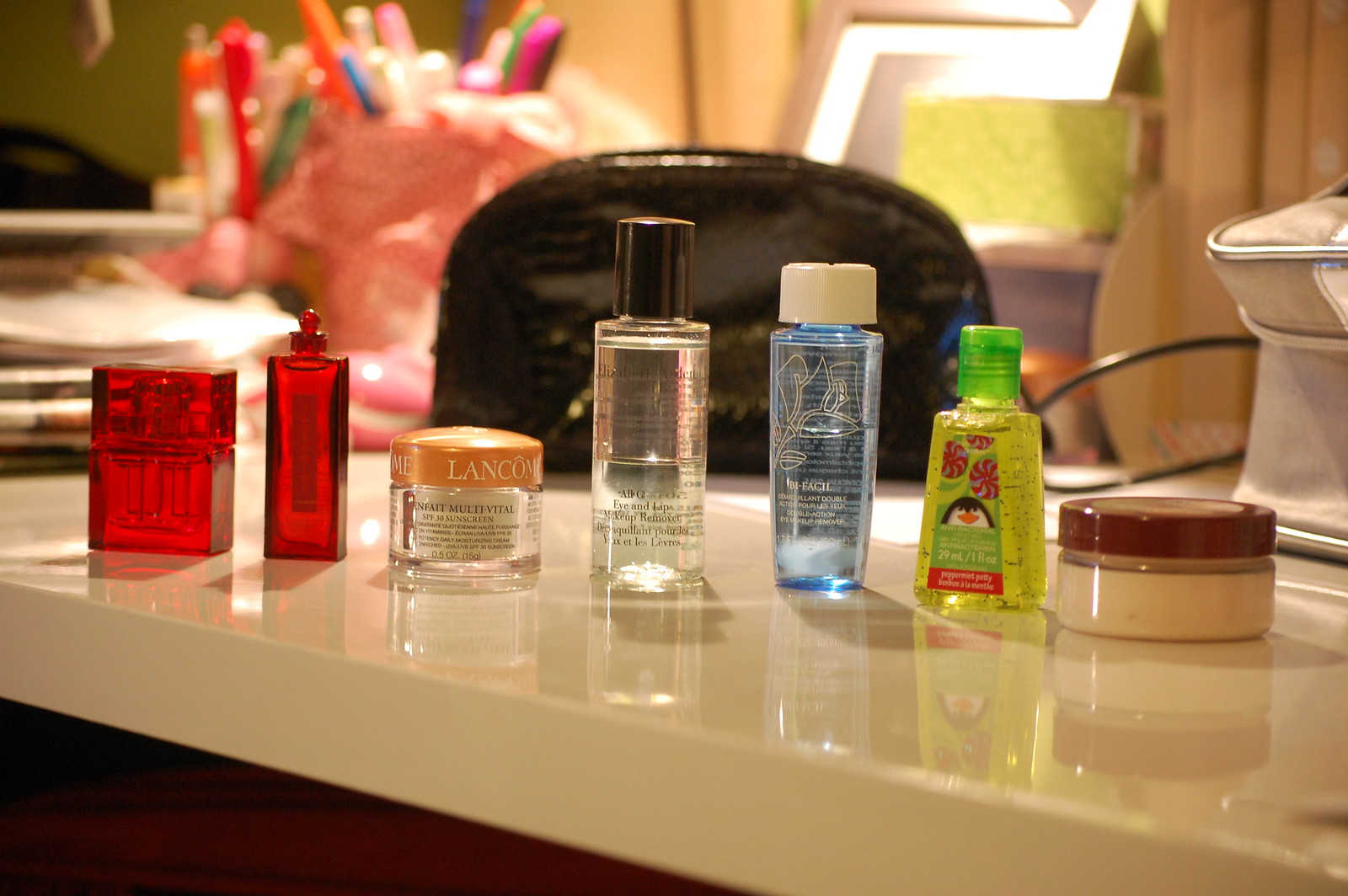This photograph captures an elegantly organized, polished stone countertop, radiating a beautiful beige hue. The gleaming surface is adorned with a diverse collection of beauty and skincare products. In the foreground, various containers filled with pens and markers are visible, adding a dash of practicality to the scene. To the far left, a stack of papers suggests a blend of utility within this refined space. Centrally located is an exquisite handbag that exudes sophistication.

The countertop is populated with an assortment of facial products and revitalizing skincare solutions. A clear bottle with a black top, designed for eye and lip care, stands prominently in the center. Next to it, a blue bottle with a white top and a red perfume bottle add vibrant touches of color. A vertical, wider red translucent dispenser and a jar with a bronze cover, indicating SPF sunscreen protection, further enrich the collection.

On the right side, various makeup and foundation jars are meticulously arranged, augmenting the aesthetic appeal. In the background, several electrical appliances are discernible, including what appears to be a curler warmer. The presence of a cord adds a hint of modernity to this visually pleasing arrangement. This captivating display might be situated in a powder room, bathroom, or even atop a kitchen breakfast bar, blending practicality with elegance.